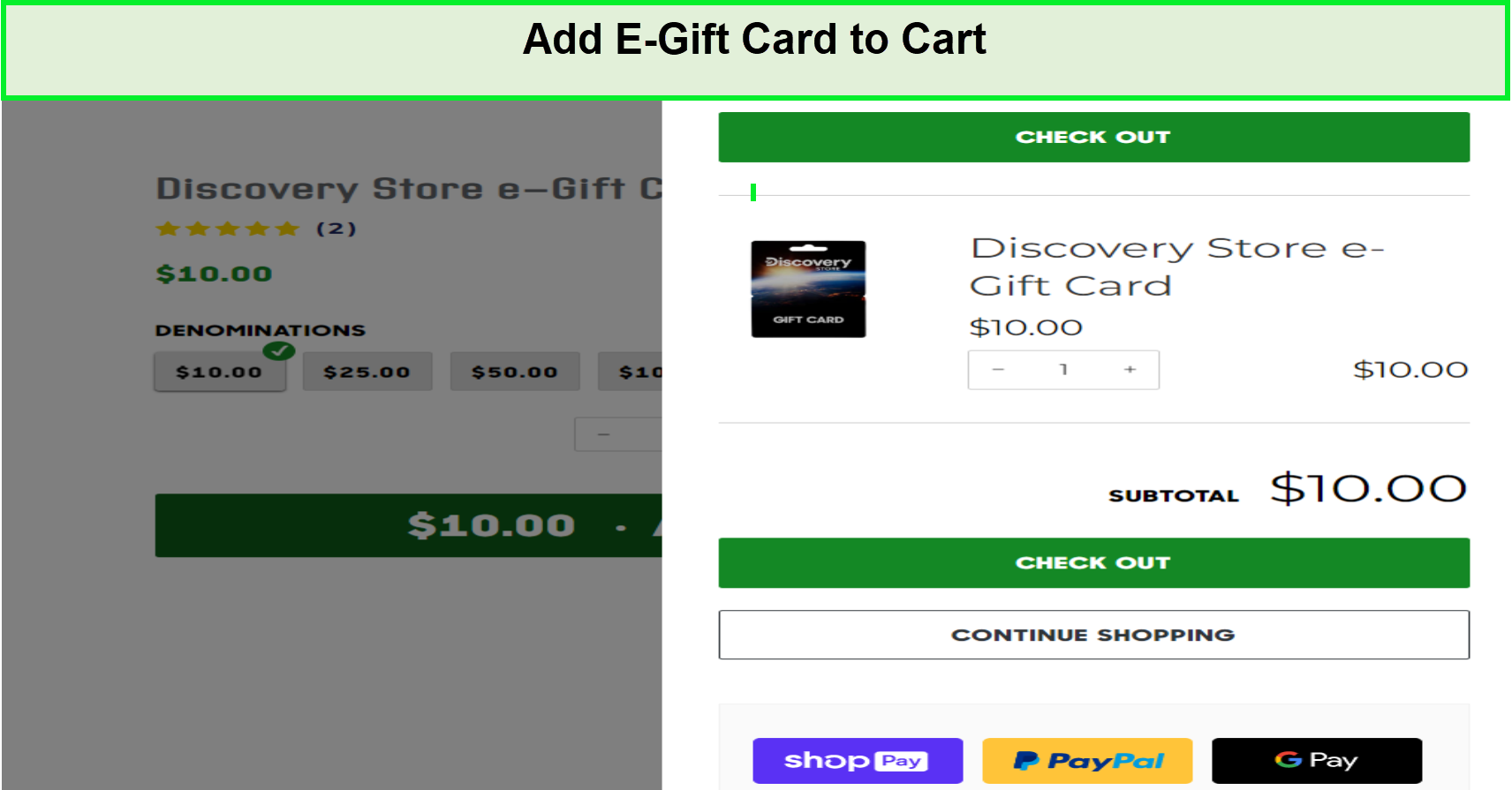This screenshot captures the process of adding an eGift card to the cart on an online storefront. 

At the top, there's a prominent dark green border around a green box with bold black text that reads "Add eGift Card to Cart." Directly below, you see a slightly grayed-out storefront section on the left half, indicating that the checkout option is currently active. The storefront section partially reads "Discovery Store eGift C," likely cut off due to the screen's proportions. This eGift card shows a 5-star rating, although it has only been rated by two customers.

The eGift card is priced at $10, displayed in green text, with options to select other denominations including $25, $50, and $100. The $10 denomination is marked with a green checkmark. Below this, a box with a minus symbol allows for adjusting the quantity.

Shifting focus to the right side of the screen, there is a green box labeled "Checkout." Below it, the text "Discovery Store eGift Card $10" is shown with a quantity of one, resulting in a subtotal of $10. An image of the Discovery eGift card is also displayed here.

Another green “Checkout” box is positioned further down, alongside a white "Continue Shopping" button. At the very bottom, alternative quick checkout options are available, including Shop Pay, PayPal, and Google Pay, indicating one-click purchasing efficiency.